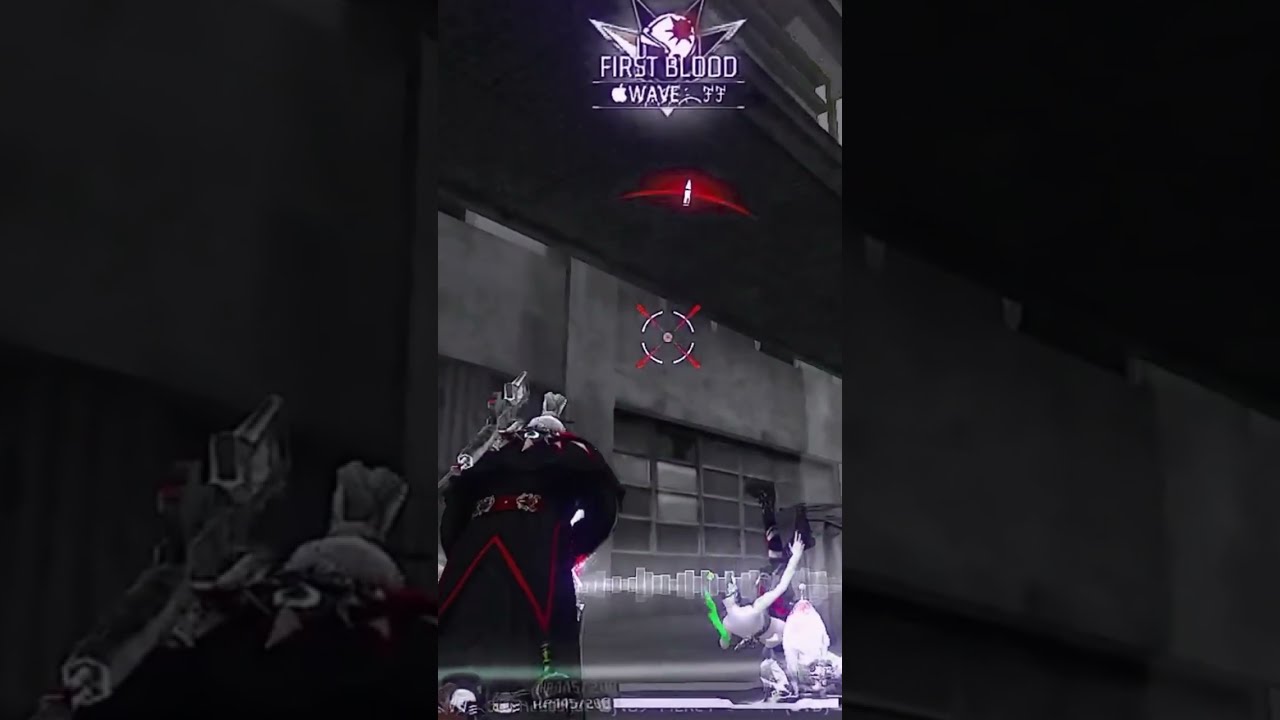This detailed image, likely a still from a video game, features a dark, fantastical scene with a central character that stands out prominently. This character, a large figure clad in a black and red robe embellished with red pinstriping, tends to dominate the visuals. The figure's head is obscured by a series of gun-like objects, contributing to the fantastical and potentially non-human quality of the character. 

The setting appears to be a warehouse or a similarly industrial environment characterized by concrete walls. There are significant symbols present – an X crossing a circle in red and white – adding to the immersive environment of the game. The overall scene is rendered primarily in dark colors such as black, white, and gray, with splashes of red and hints of purple.

In the foreground to the right, smaller characters add to the chaotic atmosphere. One figure, suggested to be a prostitute due to her attire, seems to be falling backwards with her feet up, as if she has been shot or is slipping. Another smaller figure appears man-like though indistinct in detail, enhancing the chaotic scene.

Central to the image is an imposing building with a bullseye or crosshairs symbol prominently displayed at its center, implying the viewpoint may be from a scope.

Additionally, at the top center of the image is a logo featuring a sphere with four triangles radiating outwards, flanked by the words "First Blood." Beneath this logo, in white print, is the word "WAVE" accompanied by an Apple logo. The logo area also features a red light.

Together, these elements create a vivid and dynamic scene that blends a fantastical character design with an intense, action-driven environment.